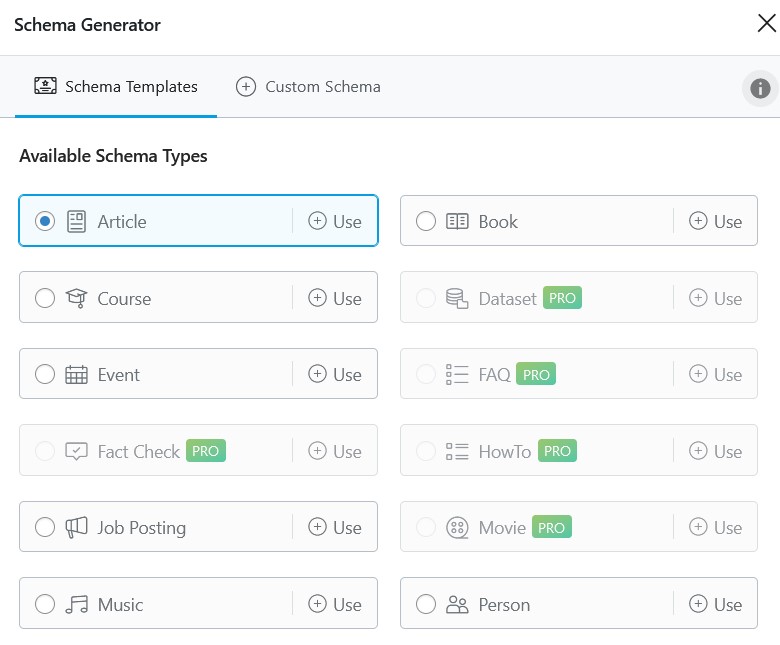In the image, we see a screenshot of a Schema Generator tool. At the top left corner, prominently displayed in bold black letters, is the title "Schema Generator". In the top right corner, there is a black 'X' button to close the window. 

Below the title, on the left side, we find the section labeled "Schema Templates" with a certificate icon next to it. Adjacent to this section is a plus symbol labeled "Custom Schema". On the far right, there is a grayish colored circle with an 'i' icon inside it, indicating additional information can be accessed by hovering over it.

Further down, there is a section titled "Available Schema Types". This section is divided into two columns, each containing six items. The left column includes:
1. Article (highlighted with a bubble to the left)
2. Course
3. Event
4. Fact Checked (marked with a green "Pro" tag)
5. Job Posting
6. Music

The right column includes:
1. Book
2. Dataset (marked with a green "Pro" tag)
3. FAQ (marked with a green "Pro" tag)
4. How To (marked with a green "Pro" tag)
5. Movie (marked with a green "Pro" tag)

The interface is designed to help users easily select and customize schemas for their specific needs.